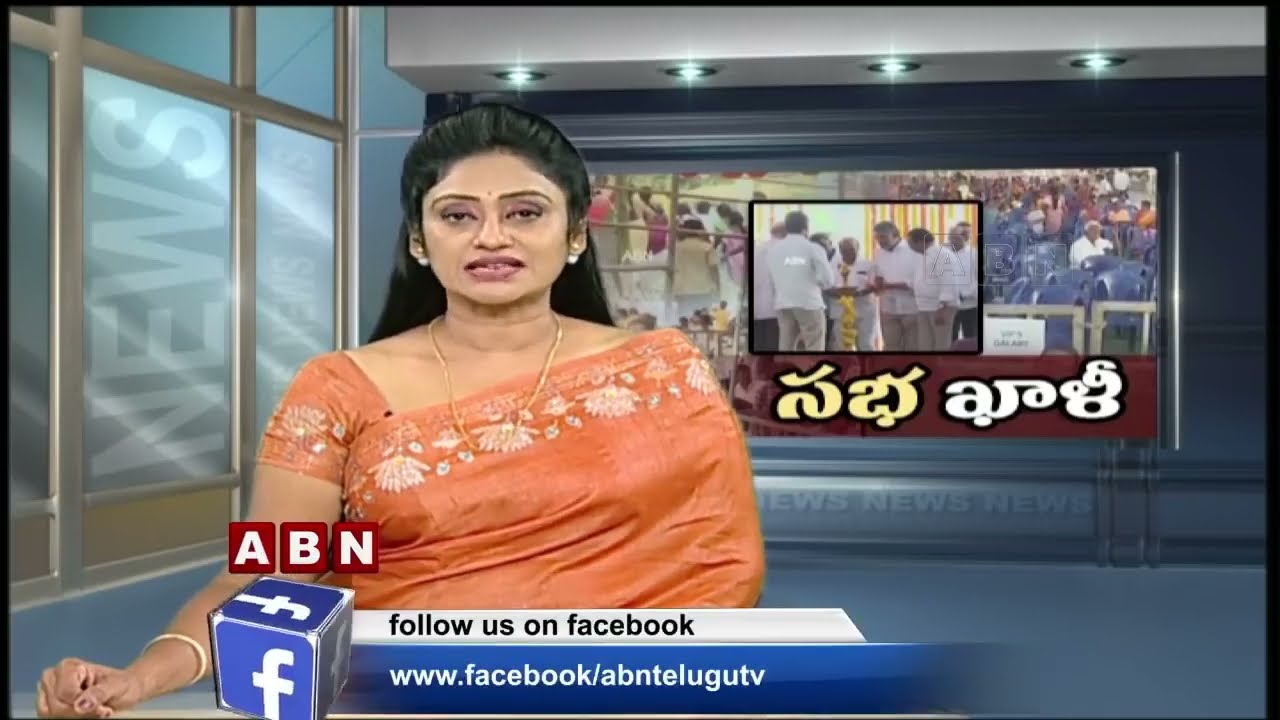The image is a screenshot from an ABN News broadcast, showing a female anchor delivering a newscast from a green screen studio. The anchor, an Indian woman, is adorned in a traditional, beautifully patterned orange sari with floral and petal designs. She accessorizes her attire with a thin gold necklace and white pearl earrings, and her hair is half-up, cascading down her back. A distinct dot adorns the center of her forehead. Behind her, the studio backdrop features digital graphics, including a fake window with the word "news" prominently displayed. There's an on-screen image showing men meeting and shaking hands, accompanied by text in an unrecognized language. The bottom of the screen displays red building blocks spelling out "ABN," along with a Facebook logo and the message, "Follow us on Facebook at www.facebook.com/abntelugutv." The anchor appears engaged in reporting the story, despite an expression that suggests a level of disinterest.